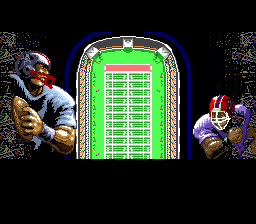In this image, we observe a pixelated depiction of a football field as viewed from a satellite or bird's-eye perspective. The green expanse of the field is bordered by pixelated sections suggesting stands filled with spectators. Flanking the field are two enlarged, detailed illustrations of football players mid-action, emphasizing the sport's dynamic nature. 

On the left, a player dons a blue jersey and a blue helmet topped with a red face guard. On the right, the opposing player wears a purple jersey paired with a red helmet featuring a white face guard. The predominant background color of the entire image is black, creating a stark contrast that highlights the green football field and the vibrant uniforms of the players. The overall composition, despite its pixelated nature, vividly communicates the essence and excitement of football.